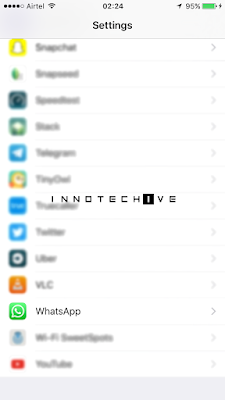**Screenshot Description:**

Captured from a smartphone with Airtel service, this image shows a screen under Wi-Fi connection, timestamped at 2:24, and indicates a battery life of 95%. The top portion features a gray bar displaying the word "SETTINGS". Below this bar, a list of app logos is visible but mostly out of focus, with notable exceptions. 

The focal point of the image is the logo for "Innotech Hive", prominently positioned in the middle of the screen. The "Innotech Hive" logo features stylized letters: the ‘O’ is a square, and the ‘I’ in "Hive" is a black box with a white ‘I’. The remaining letters are in black text.

Background app logos are partially visible through the blur: 

- At the top, the Snapchat logo is identifiable.
- Near the center, the Telegram logo can be clearly read.
- Below the "Innotech Hive" logo, the Twitter logo is discernible.
- Further down, the WhatsApp logo is seen.
- At the very bottom, the YouTube logo is visible.

Other app logos remain blurry and indeterminate.